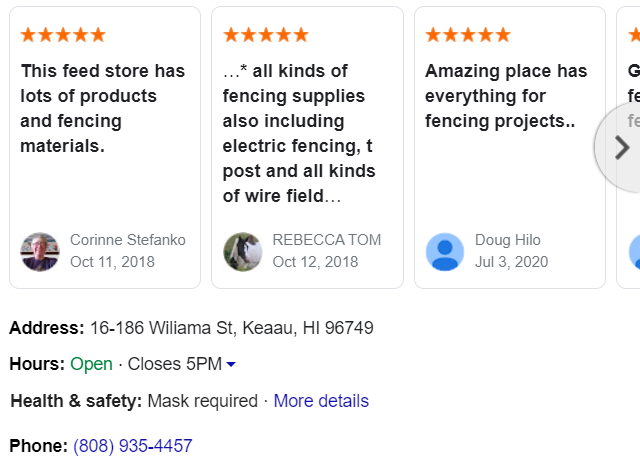The search results display three highly-rated reviews for a feed store located at 16-186 William Street, Keoma, Hawaii, 96749. All three reviews praise the store's extensive selection of fencing materials.

1. **Corrine Stefanko** - *Posted on October 11, 2018*. Avatar: A small image of herself. 
   - **Rating**: ★★★★★ (5/5)
   - **Review**: "This feed store has lots of products and fencing materials."

2. **Rebecca Tom** - *Posted on October 12, 2018*. Avatar: A picture of her cat.
   - **Rating**: ★★★★★ (5/5)
   - **Review**: "All kinds of fencing supplies, including electric fencing, posts, and various wire options."

3. **Doug Hilo** - *Posted on July 3, 2020*. Avatar: A generic blue background with a blue person figurine.
   - **Rating**: ★★★★★ (5/5)
   - **Review**: "Amazing place has everything for fencing projects."

**Store Details**:
- **Address**: 16-186 William Street, Keoma, Hawaii, 96749
- **Phone Number**: 808-935-4457
- **Hours**: Open, closes at 5 p.m.
- **Health and Safety**: Masks required. [More details]

This store is highly recommended for its wide range of fencing supplies, evident from the five-star ratings and positive feedback from customers.